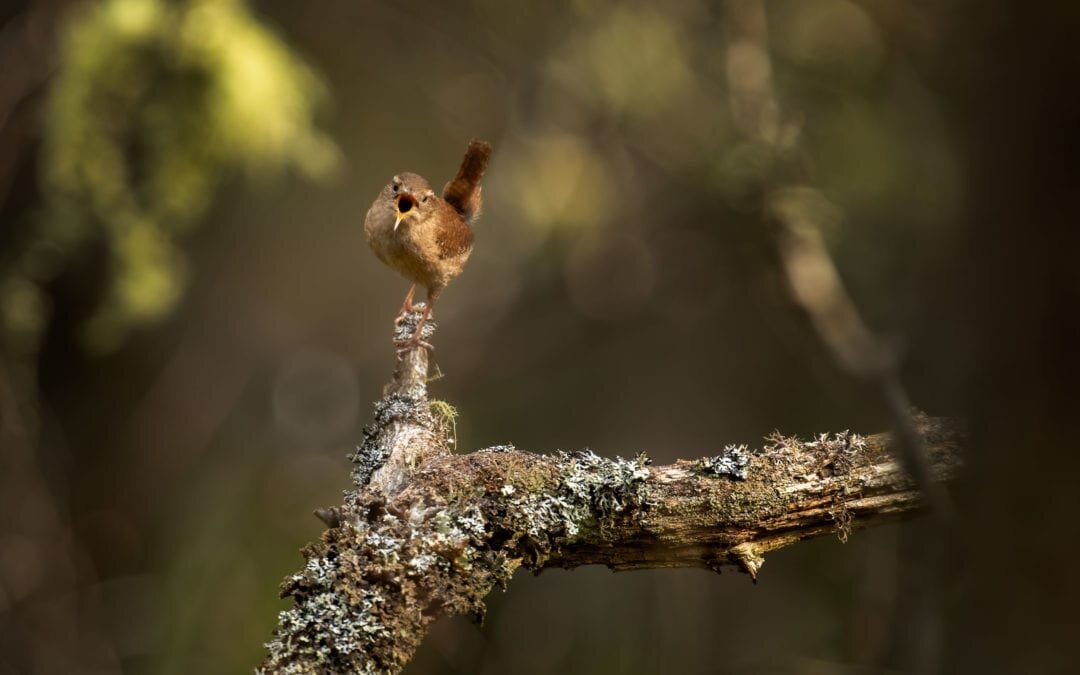In this photograph, taken in an outdoor setting with a deliberately blurred background, the main focus is a detailed, close-up view of a bird perched on a tree branch. The background, a mix of indistinct greens and yellows, frames the scene with a soft, natural glow. The branch, prominently featured, is predominantly brown with patches of green moss scattered throughout, revealing the textured grooves of the bark. The branch extends diagonally from the bottom of the frame, splitting into a longer piece to the right and another rising slightly to the left.

Perched on the upright portion of the branch is a small, brown bird with a strikingly vivid yellow beak. The bird's eyes are looking directly at the camera, and its mouth is wide open, capturing a moment that suggests chirping or singing. White, bushy feathers adorn its eyebrows, and its tail feathers are a dark brown. The image's composition draws immediate attention to the bird and the intricately detailed branch, emphasizing the natural and serene beauty of the scene.